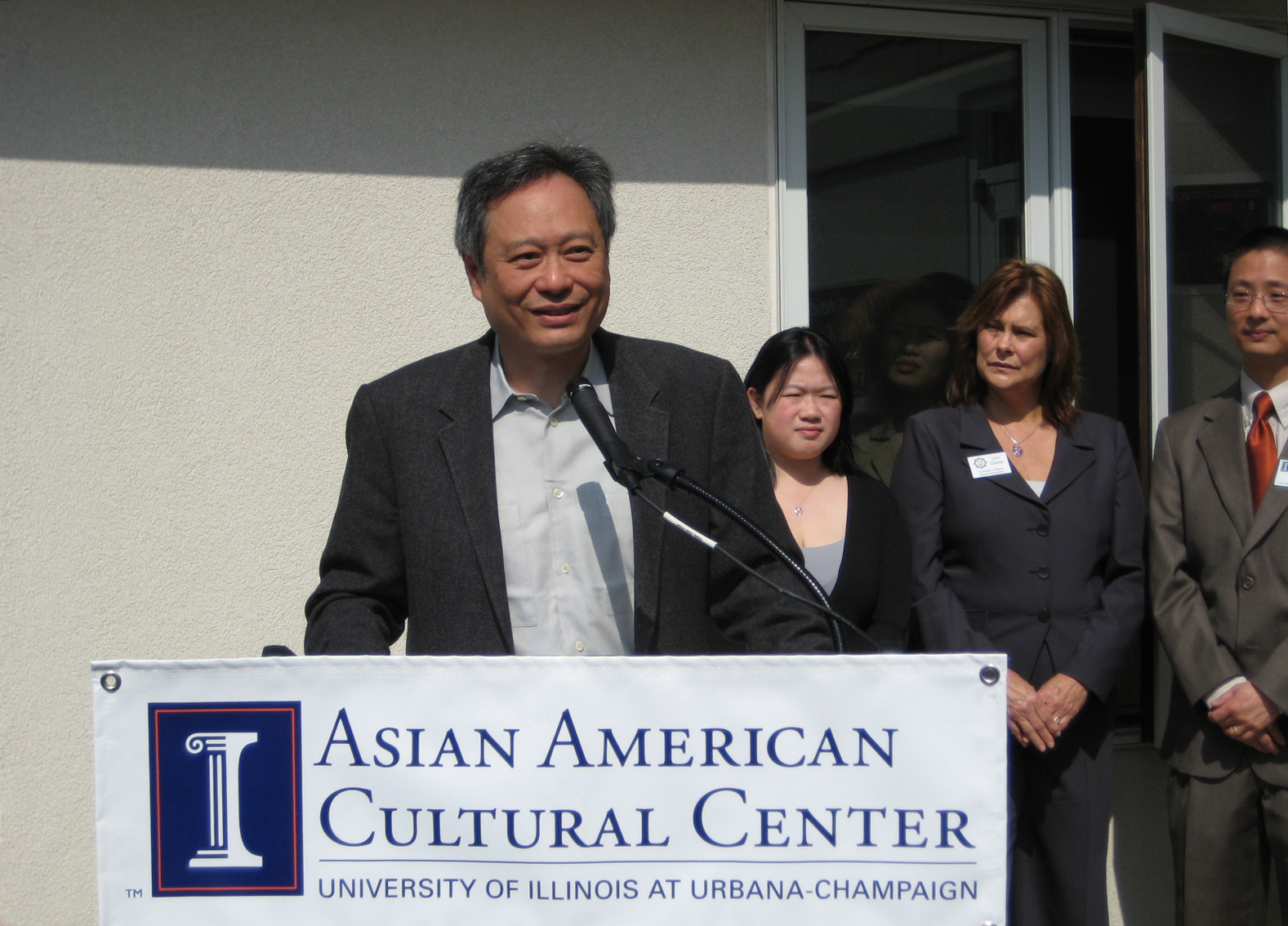The photograph captures a professional event at the University of Illinois at Urbana-Champaign. Central to the image is an Asian gentleman, possibly 50 to 60 years old, standing on a stage behind a podium, addressing the audience with a smile. He is dressed in a white t-shirt, black jacket, and speaks into a black microphone attached to a stand. The podium displays a white banner featuring the blue and white logo of the Asian American Cultural Center, bordered in orange, with the center's name written in blue text.

Surrounding him, there are three formally dressed individuals in the background—a man and two women. The man on the right is wearing a brown suit jacket, red tie, grey pants, and glasses, with a name card on his chest. The central female figure is adorned in a black jacket and a necklace, also bearing a name card, while the other woman, with black hair, is dressed in a black top. The backdrop of the photograph reveals a half-white wall and a glass door to the right. The overall ambiance is professional and engaging, highlighting a significant moment for the Asian American Cultural Center.